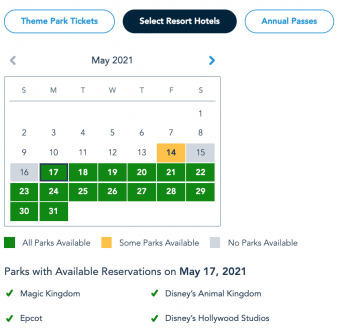This image is a screenshot from an unspecified source, providing information on theme park reservations for various dates in May 2021. The top of the image features options for "Theme Park Tickets," "Select Resort Hotels," and "Annual Passes," with the "Select Resort Hotels" section currently highlighted. A calendar for May 2021 is displayed, showing different color-coded availability statuses for park reservations: May 14th is marked in orange, indicating some parks are available; May 15th and 16th are shaded in gray, denoting no park availability; and May 17th through 31st are in green, signifying all parks are available. 

A legend below the calendar indicates the meaning of the colors: green for all parks available, orange for some parks available, and gray for no parks available. There is further clarification that on May 17, 2021, all four major Disney parks—Magic Kingdom, EPCOT, Disney's Animal Kingdom, and Disney's Hollywood Studios—have available reservations. 

The image is strictly informational and contains no photographic or illustrative elements. There are no depictions of people, animals, birds, plants, flowers, trees, buildings, automobiles, motorcycles, bicycles, or airplanes.